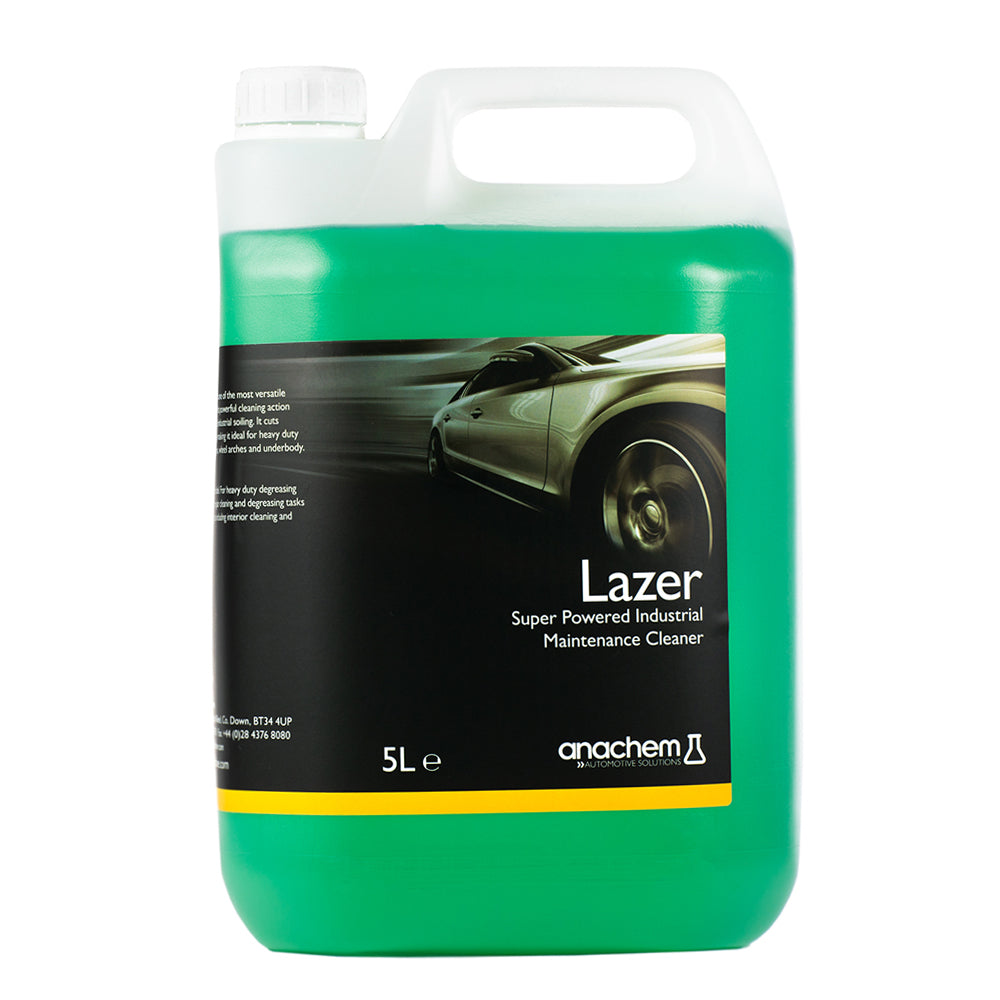The image features a large, clear plastic jug designed for car maintenance, filled almost to the top with a vibrant lime green liquid. The jug has a flat bottom with gently curved sides that rise straight up, culminating in a large, rectangular plastic handle with an oval-shaped hole on the right. To the left of the handle, there is a white screw cap. The jug prominently displays a black label that wraps around from the left side, adorned with a photograph of a silver car in motion, wheels spinning, located mainly on the right side of the label. The navigable text reads "LASER Super Powered Industrial Maintenance Cleaner" in white, followed by "5L" which denotes its five-liter capacity. The manufacturer is "ANACHEM Automotive Solutions," indicated by white text along with a small logo of a science laboratory beaker. The label also features a yellow stripe at the bottom and some additional, less legible text. The image has a clean, white background, making the details of the jug and its label highly visible.